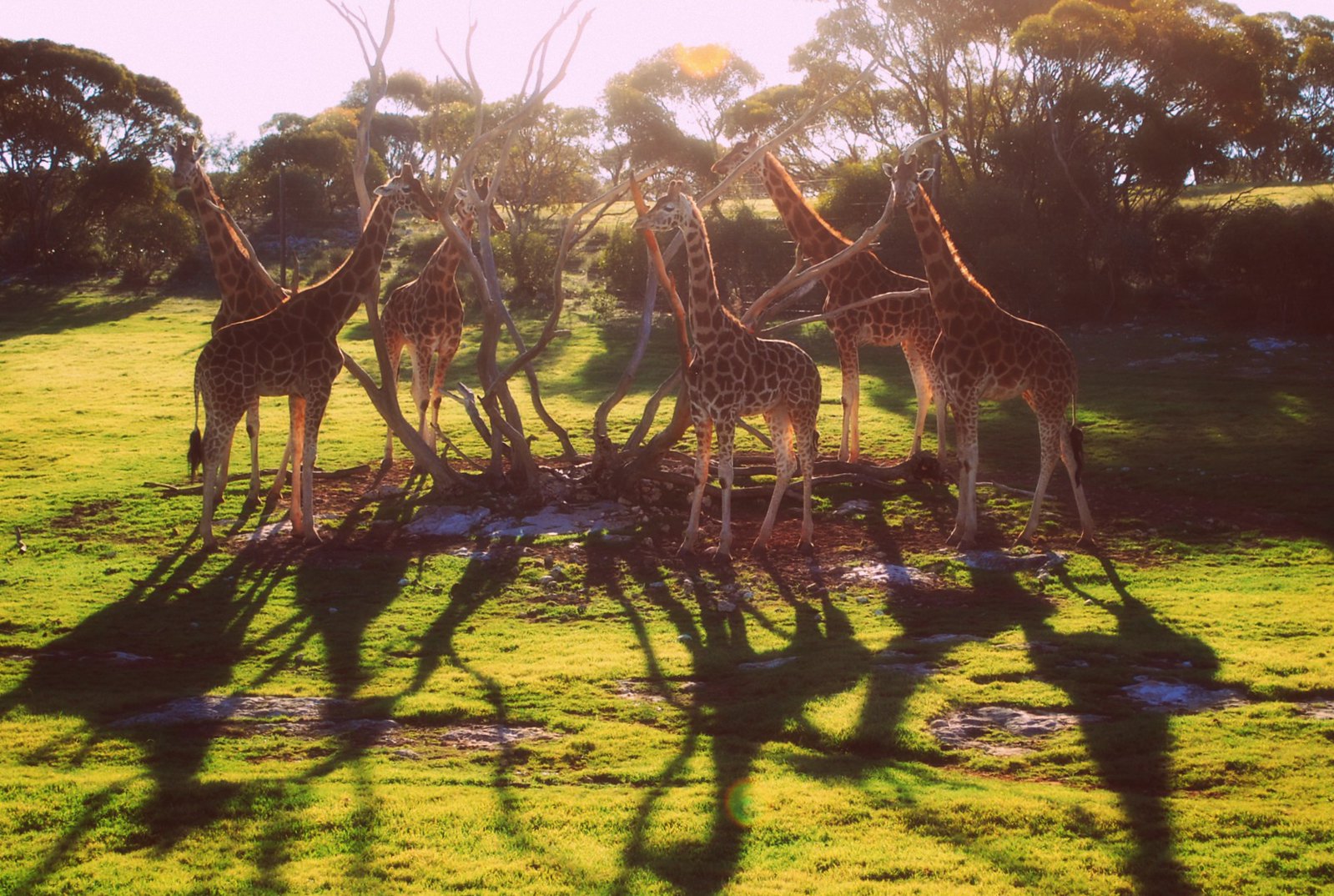In this outdoor scene, the sky is a light blue mixed with purple hues, suggesting that the photo was taken around sunset, as the long shadows of the giraffes are visible on the ground. In the background, a line of tall, full trees stretches across the horizon, just above a shallow, grassy hill. Closer to the foreground, a herd of giraffes is gathered in a circle around a central area featuring leafless trees with long, visible roots, possibly sticking out of the ground. Under these trees, there is a mud puddle surrounded by dirt, contrasting with the grassy field that spreads out across the rest of the scene. The giraffes, appearing relatively young and not very tall, all face toward the central mud and tree area. Broken patches of grass and shadows on the ground add texture to the landscape, enhancing the sense of a natural grassland environment akin to the African plains.